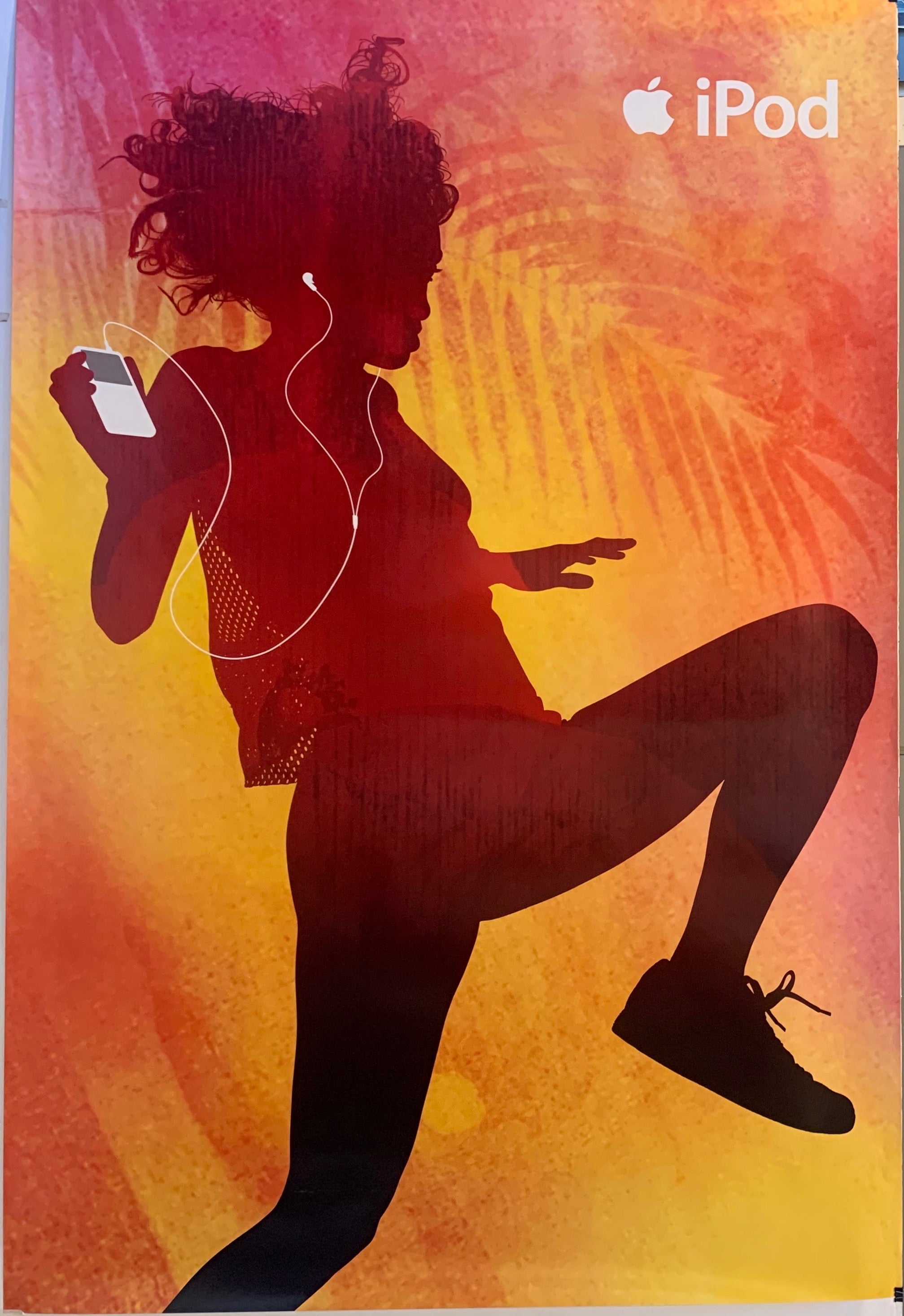This vibrant iPod advertisement poster prominently features the Apple logo in the upper right corner alongside the word "iPod" written in white. The background is a stylized tropical theme awash with shades of pink, yellow, and orange, resembling a picturesque sunset. A faintly etched palm leaf adds to the tropical ambiance. At the center, a silhouetted woman dances energetically, her figure defined against the colorful backdrop. She has curly hair and is depicted with one leg lifted and bent at the knee, wearing black sneakers. The woman is equipped with wired headphones and holds an iPod in her right hand, with the headphone cord visibly trailing from the device. Her dark silhouette contrasts sharply with the vivid background, giving the impression of movement and joy as she dances in the sunset.